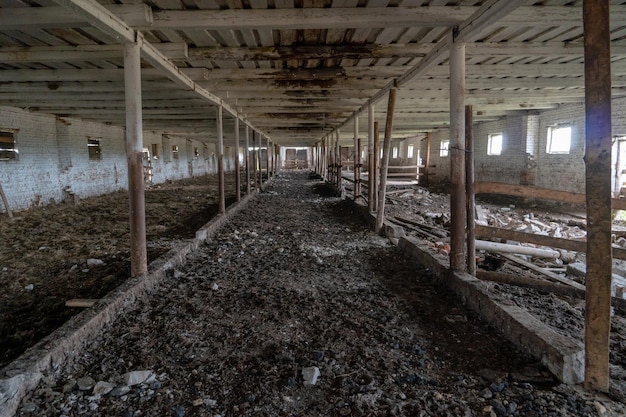The photograph depicts a long, dilapidated, and abandoned building, possibly once a chicken coop or some form of farm structure. The structure features a low, decaying roof, marked by large brown stains suggesting rust or water damage. The interior extends down a central gravel path, bordered by chunky blocks or stones, leading to barely visible double doors at the far end. 

Each side of this path is flanked by round metal or stone pillars supporting the deteriorating ceiling, which consists of either stained metal sheets or wooden slats. The walls, constructed of stone or perhaps whitewashed wood, are punctuated by square windows. On the right side, windows allow sunlight to stream in, while those on the left remain shrouded in darkness, possibly boarded up or simply shadowed. The ground is strewn with debris and dirt, indicating many years of neglect and disuse.